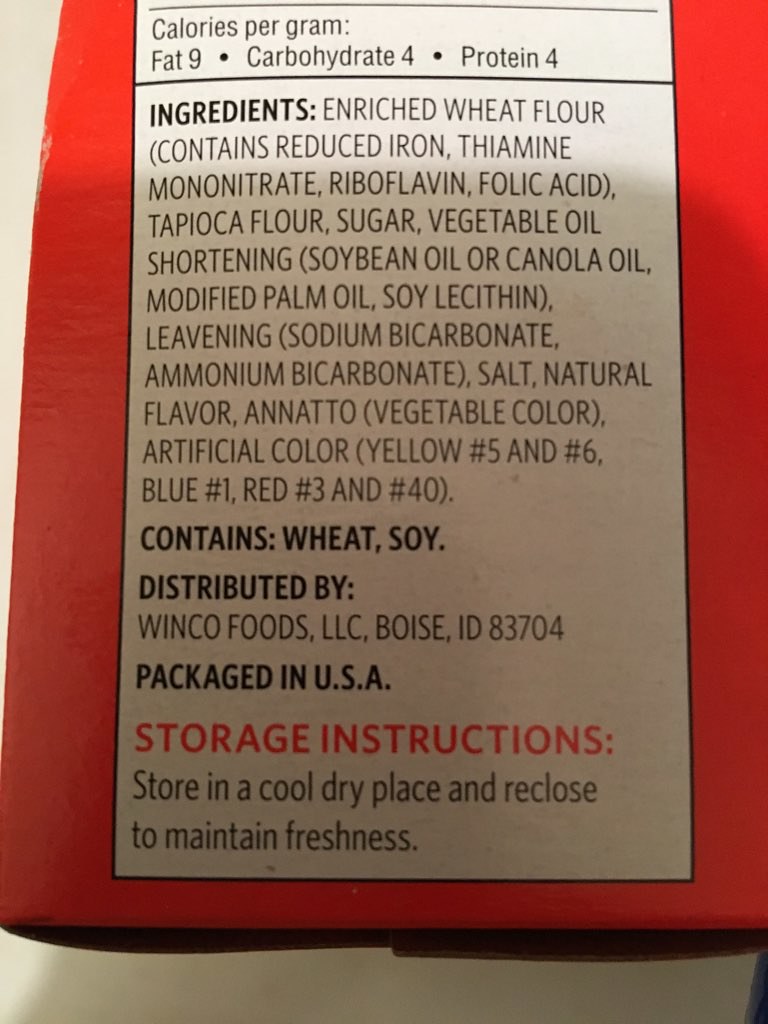The image shows a detailed photograph of the ingredients list on the back of a food product packaging. The ingredients are displayed inside a white rectangular box which is set against a red background that wraps around the entire packaging. The product contains enriched wheat flour, assorted oils including canola and palm oil, sugar, salt, natural flavor, and multiple artificial colors such as Yellow No. 5 and 6, Blue No. 1 and 3, and Red No. 40. It is indicated that the product contains wheat and soy, and has enrichment additives like thiamin, mononitrate, riboflavin, folic acid, and reduced iron. The packaging advises storing the item in a cool, dry place and re-closing it to maintain freshness. The box also shows distribution details stating it is distributed by Paxigen USA, and the flaps at the bottom of the box suggest it is a cardboard box, likely for a product such as bread or cereal.